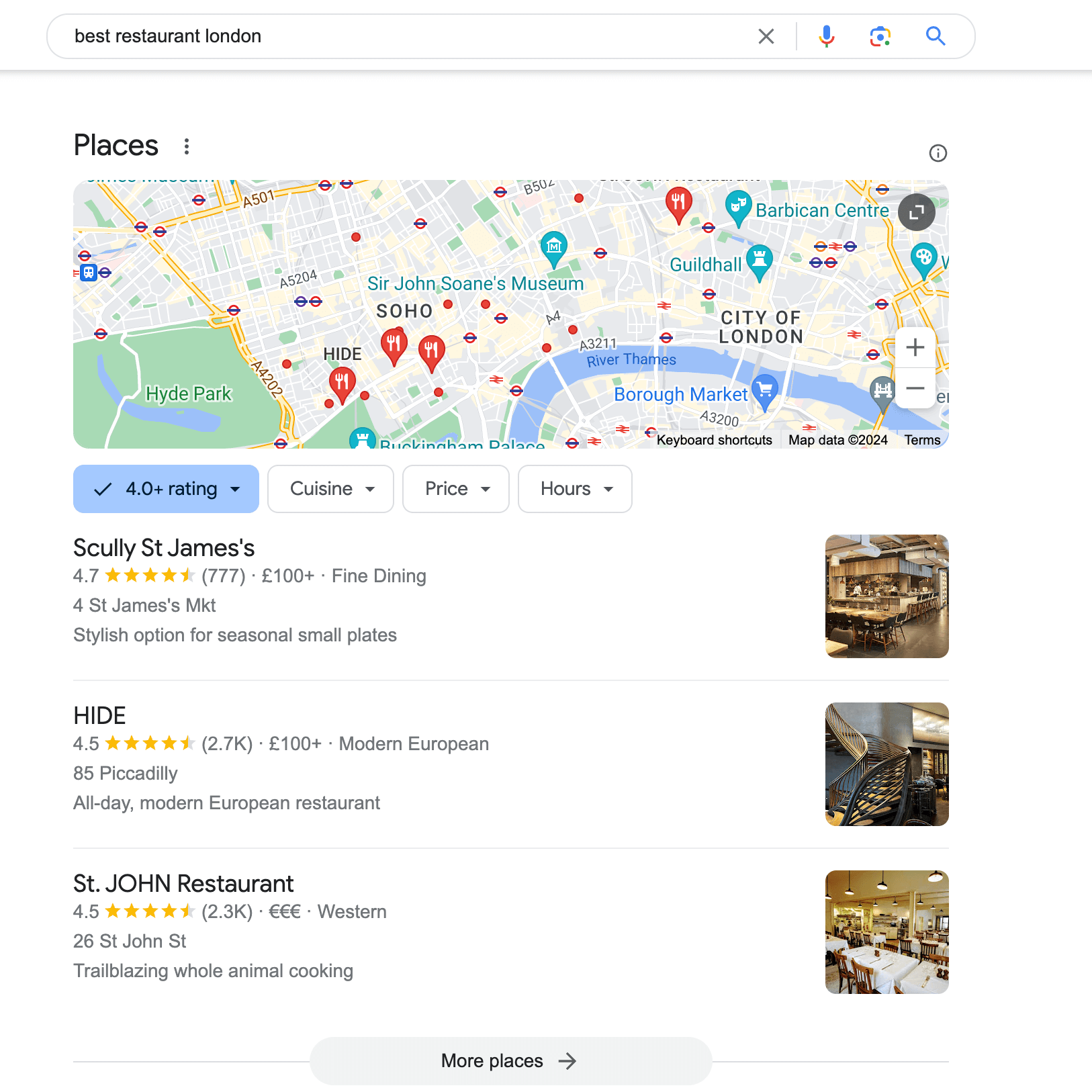The image depicts a Google search being conducted on a tablet with the query "best restaurant London" typed into the search bar at the top. The search bar is a long oval strip with a white background and the text is displayed in black Arial font. Towards the right of the search bar is a gray 'X' icon followed by a gray line divider. Adjacent to this, the Google voice search microphone is visible, adorned with the traditional Google colors. Additionally, there is an option for an image search with an icon in Google colors, and towards the right end is a blue magnifying glass icon.

Below the search bar, the interface is divided by a shadowy-effect gray line. On the top left, the word "Places" is displayed in black text. To the right of it are three vertical black dots, suggesting further options. The screen then showcases a rectangular map area with rounded corners. Beneath the map, there is a filtering option that says "4.0+ rating" with a dropdown symbol, highlighted in blue to indicate it is selected, with a checkmark to its left. To the right of this filter, there are three filter options with dropdown menus: "Cuisine," "Price," and "Hours," each displayed in black font on a white background with a light gray border.

The first listing displayed is for "Scully St. James's." On the right side of the listing, there is a small image of the establishment. Below the restaurant name, in smaller gray lettering, it shows a rating of 4.7 out of 5, indicated by four and a half stars being highlighted. To the right of the rating, it states "(777)" to denote the number of reviews. Following this, there is a bullet point followed by a British pound sign and "100+," indicating the price range. Another bullet point follows, labeling the restaurant as "Fine Dining."